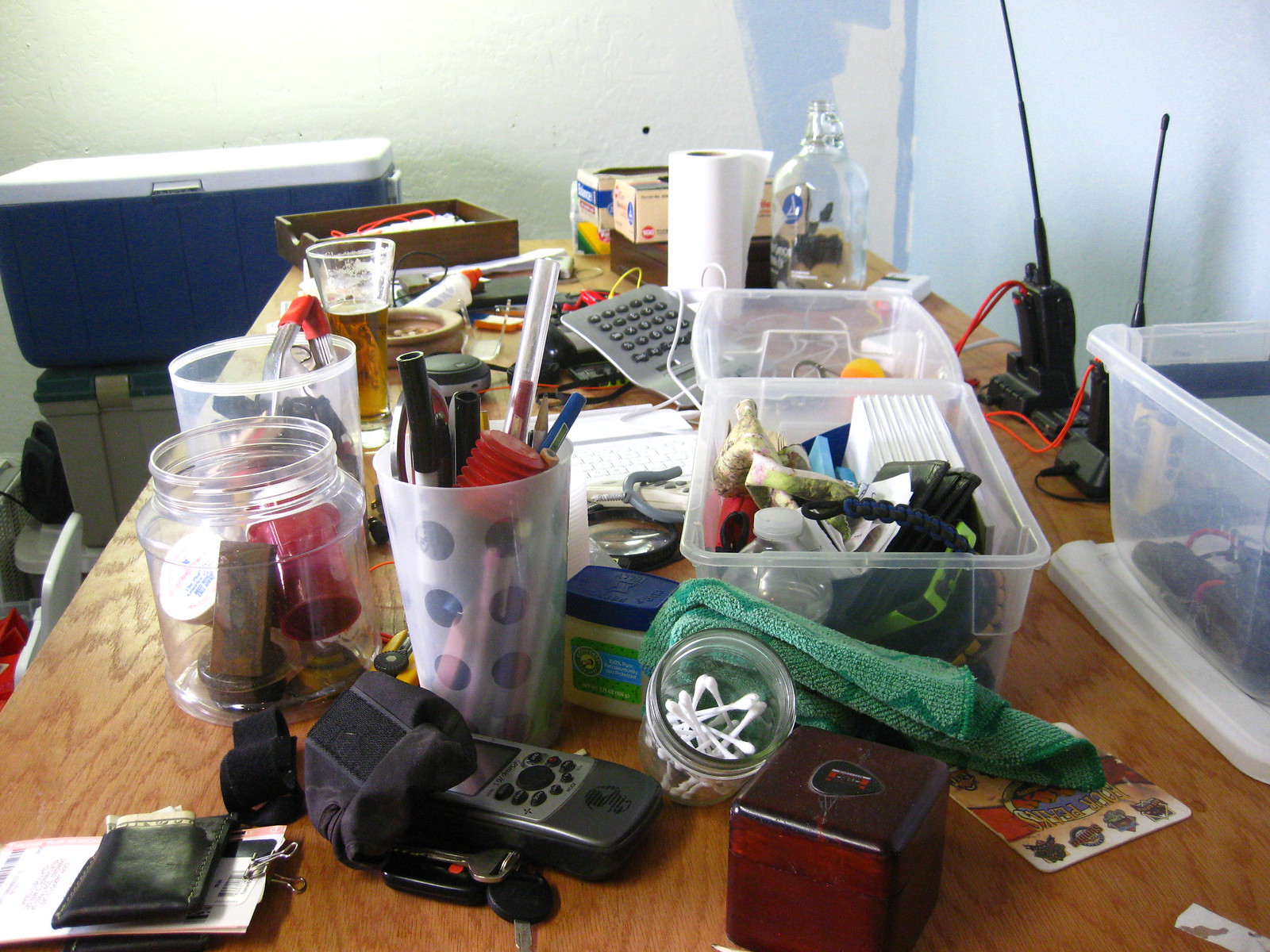A cluttered wooden table spans the entire foreground of the photograph, covered with a myriad of assorted items as if someone has emptied a junk drawer onto it. Starting from the left, a wallet partially revealing some money sits atop a stack of receipts. Adjacent to the wallet, a remote, a car key, and a dark reddish cube add to the disarray. A small glass jar containing Q-tips stands beside a green washcloth.

Further along the table, a plastic tub brimming with miscellaneous objects, including what appear to be white cards, occupies a central position. Next to it, a plastic cup brimming with pens is positioned alongside a glass jar holding a red plastic item, possibly a spool. A silver calculator and a jar of Vaseline are also visible in this clutter. Another plastic cup sits behind these items.

To the right side of the table, a plastic bin with its lid removed partly extends out of the frame. A pair of black walkie-talkies with extended antennas and dangling red cords stands upright behind the bin. At the far end of the table, a roll of paper towels stands upright next to a white jar that tapers at the top.

In the background, to the left of the table, a plastic file box supports a large blue cooler with a white lid. The room's wall is in the midst of being painted, showcasing a transition from white beige on the left to light blue on the far right, with an incomplete section of a slightly darker blue paint adjacent to the lighter shade.

The overall impression is one of a chaotic assortment of everyday objects strewn haphazardly across the table, creating a visually overwhelming scene.